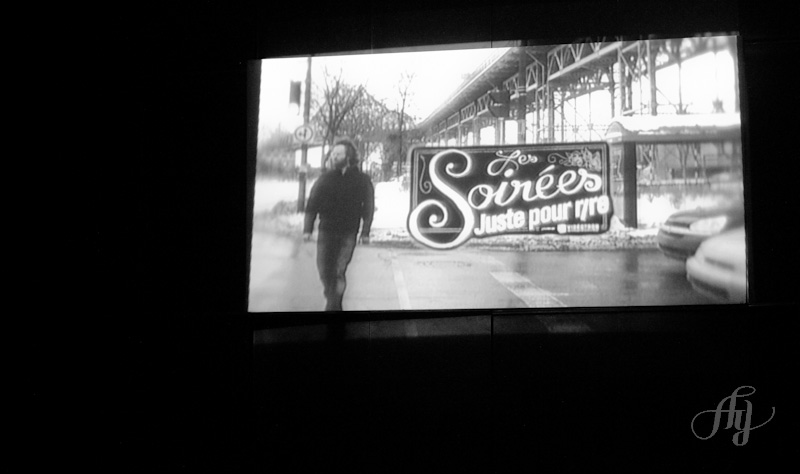The image is a rectangular black and white photograph, potentially of a television screen, taken in a dark room. The majority of the image's background is black, with a prominent screen situated in the upper third on the right-hand side. The screen captures a grainy black and white street scene: a bearded man in his 30s, wearing a long-sleeved coat and jeans, crosses a snow-dusted crosswalk. He looks to his left, away from the camera. To his right, the headlights of two stopped cars—one lighter and one darker—are visible, though the make of the cars is indiscernible. 

Directly in front of the man and spanning the middle of the image is a banner with a black background and elegant, French script reading "Les Soirées Juste Pour Rire." Behind the man, there is a clear glass bus stop, and above, an elevated roadway or subway track. Further in the distance, a large bridge is visible, suggesting the presence of a river or another major roadway beneath.

In the bottom right-hand corner of the image, a small, curvy logo can be seen, reading "FYY," presumably the signature or watermark of the photographer or creator. Although the scene is bright, indicating a sunny day, the black and white format makes it difficult to ascertain specific weather conditions.